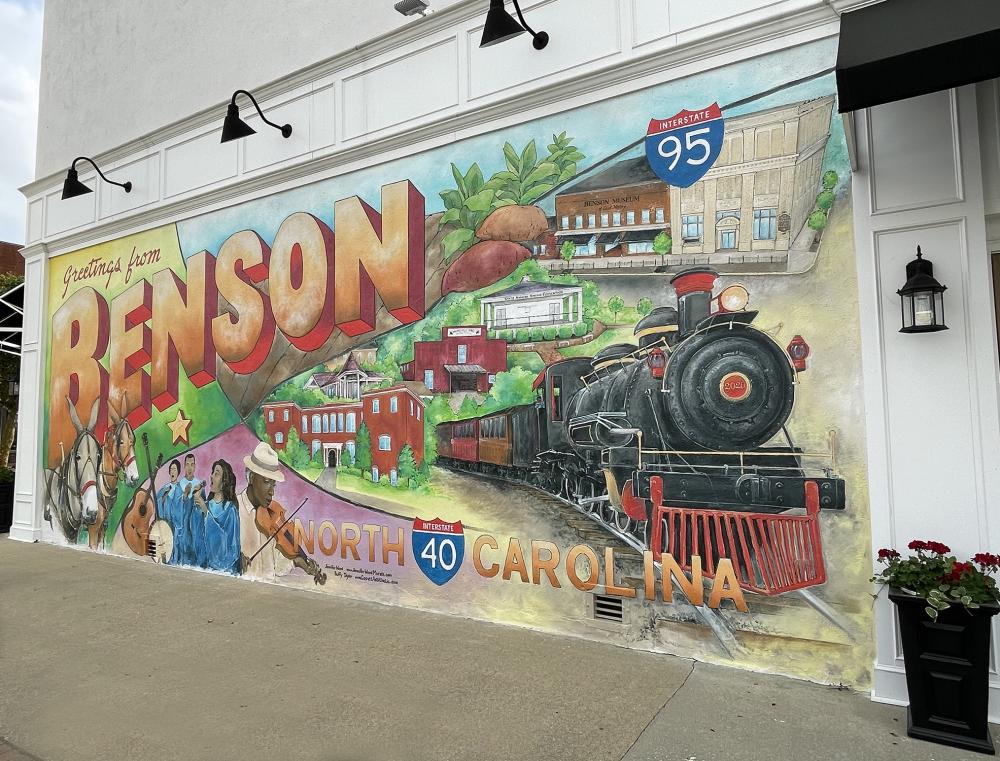This image showcases an intricately designed mural on the side of a white building, accentuated by three black lamps hanging above it. Dominating the upper-left corner of the mural are the words “Greetings from Benson” in vibrant, artistic letters, with "Benson" prominently displayed in large, striking orange letters. Beneath the "B," there are two horses—a brown one and a gray one. The mural also features a diverse array of elements: under the letter "N," set against a green background, is a bright yellow star, and directly below this star, three individuals dressed in blue choir gowns stand out. To their left, musical instruments, including a guitar and a banjo, are depicted, alongside a man in a beige outfit playing a violin. The lower section of the mural prominently displays the phrase “North Carolina” along with a shield graphic indicating Interstate 40. Above the word "Carolina," a black train with a red grill faces outward, and above the train, another shield marks Interstate 95. Additionally, the mural encapsulates elements of Benson’s local life, including houses, trees, and various types of people, providing a vibrant snapshot of the community. There are also visual details outside the mural, including a lantern and a rectangular vase filled with red roses, adding an element of charm to the mural's immediate surroundings.